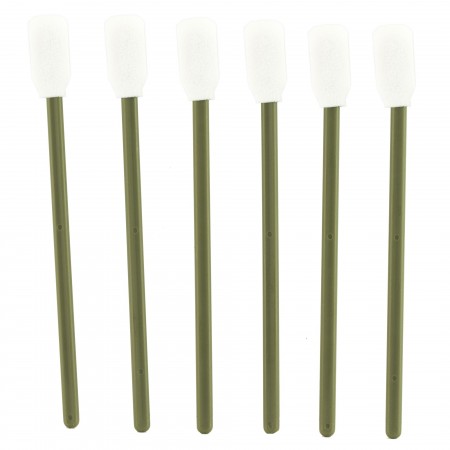The image depicts six identical objects, all standing upright in a vertical orientation. These objects resemble long, olive-green sticks with a glossy white cap at the top, similar in appearance to Q-tips but without the fuzzy ends—more akin to a matchstick with a white tip. Each stick is evenly spaced, taking up nearly the entire frame of the image and set against a plain white background with no text or other elements. The overall impression is of a product shot, potentially for a website, highlighting these sleek, uniformly arranged objects.